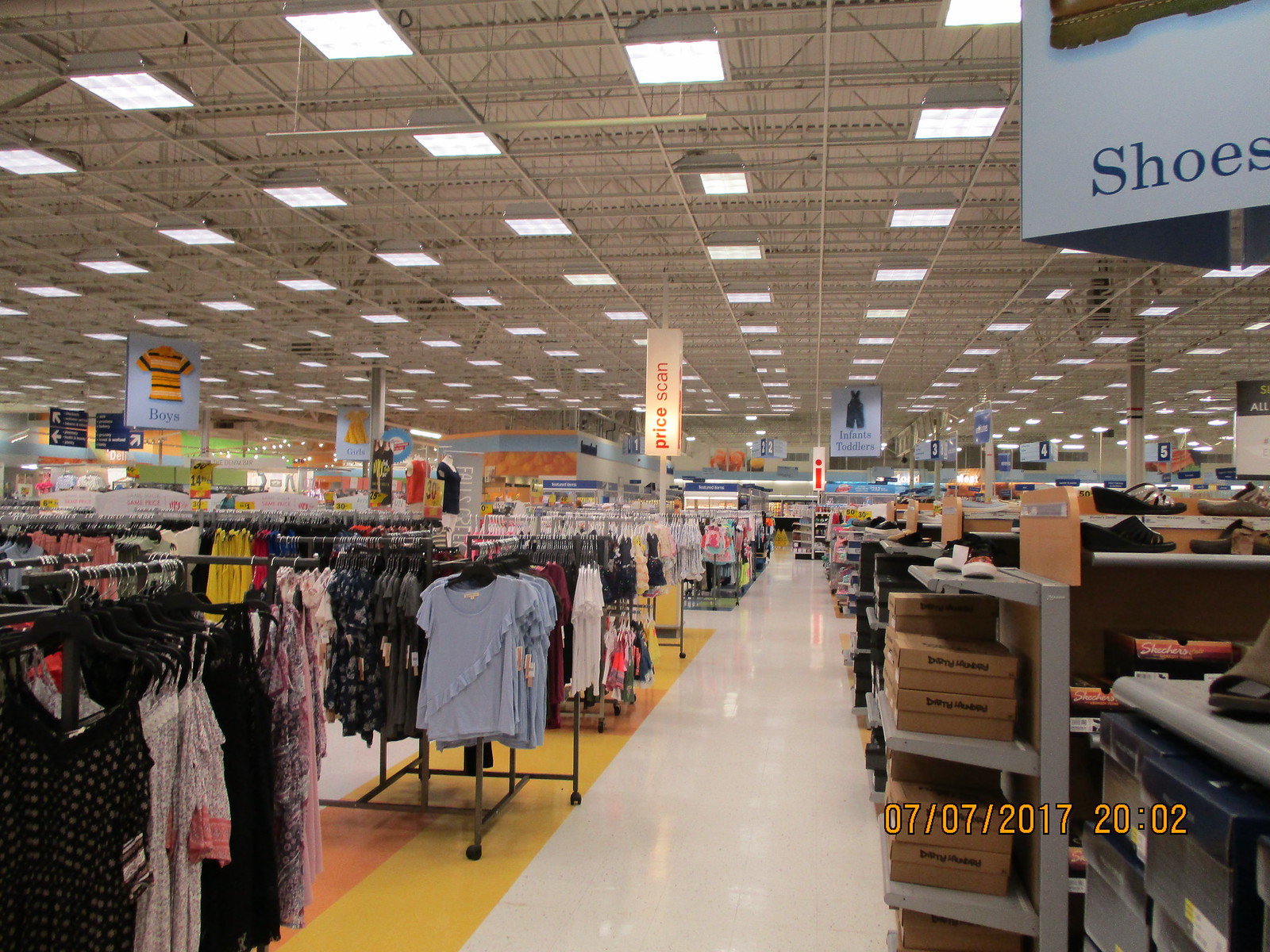This image depicts the interior of a sprawling department store, likely a Target, characterized by an open layout and a warehouse-like atmosphere. Dominating the left side are racks of women's clothing, notably blouses, neatly arranged on hangers. The flooring features an off-white color with some yellow squares framed by orange accents, contributing to the store's vintage feel. Prominent overhead signage includes a blue "shoes" sign on a white background to the right, marking aisles filled with shoes displayed both in boxes and on racks for easy viewing. Another sign reads "price scan," indicative of the store's familiarity. The ceiling lacks traditional tiles, exposing metal supports and scaffolding, with fluorescent lights providing ample illumination. There's a timestamp in the bottom right corner, marking the image as taken on July 7th, 2017, at 8:02 PM, further cementing its lived-in authenticity.